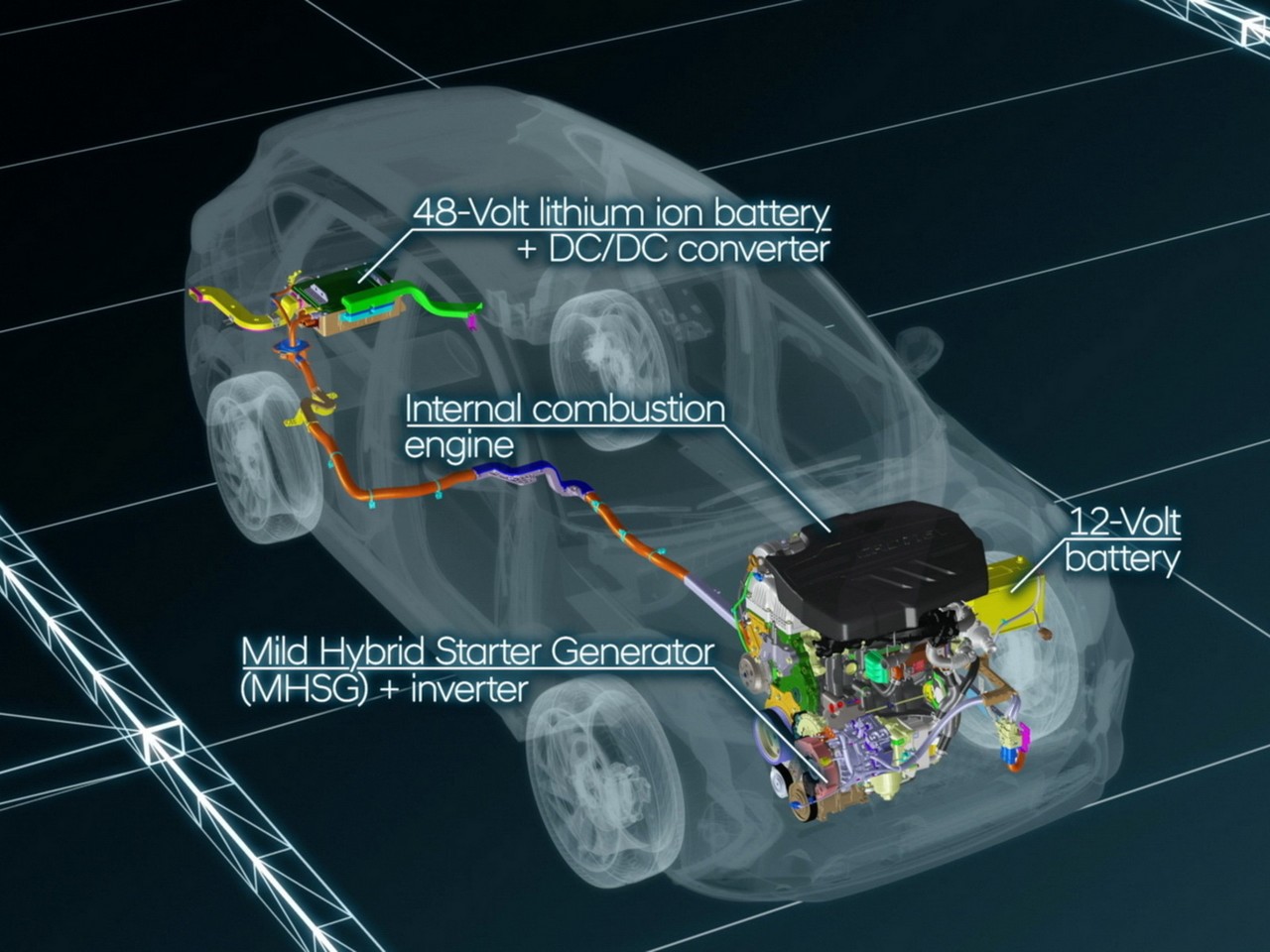The image showcases a detailed digital 3D model of the internal structure of a normal-sized four or five-seater car, resembling an x-ray view. The semi-transparent depiction reveals the car's tire base and entire inner framework, making the structure visible like a skeletal outline. The car is overlaid on a grid background, with various colorful lines and labels pinpointing key components. The front of the car highlights the engine, featuring a yellow part labeled as a 12-volt battery. Nearby, another label points to a component marked "mild hybrid starter generator (MHSG) plus inverter." Extending from the engine area to the car's rear is a coil, indicating the internal combustion engine. Positioned at the back, the image labels a 48-volt lithium-ion battery connected to a DC/DC converter. Each car part is distinctly color-coded in hues of yellow, green, blue, pink, orange, and purple, facilitating a clear understanding of the vehicle's intricate makeup.